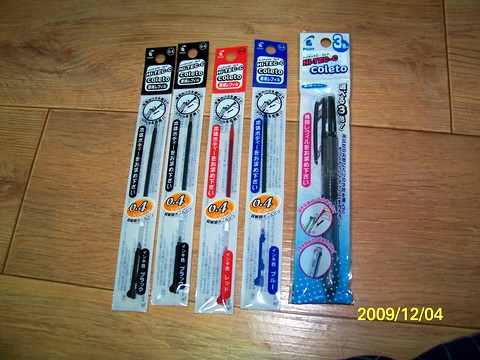The image depicts various art supplies neatly arranged on a light tan wooden floor with large sections. Dominating the scene are five packages, still in their plastic wrappers, showcasing pen refills and a multi-color pen. The refills come in black, red, and blue, with two black refills on the left, a red one next to them, and a blue one to the right. To the far right is a distinctive package containing a multi-color pen designed to hold these refills. All the packages display the Pilot logo and Japanese or possibly Korean characters, indicating their origin. The top of the pen's package is labeled "Hi-Tec C Coletto" in blue and white. At the bottom right of the image, the date "2009/12/04" is visible in yellow numerals and slashes, marking when the photograph was taken.